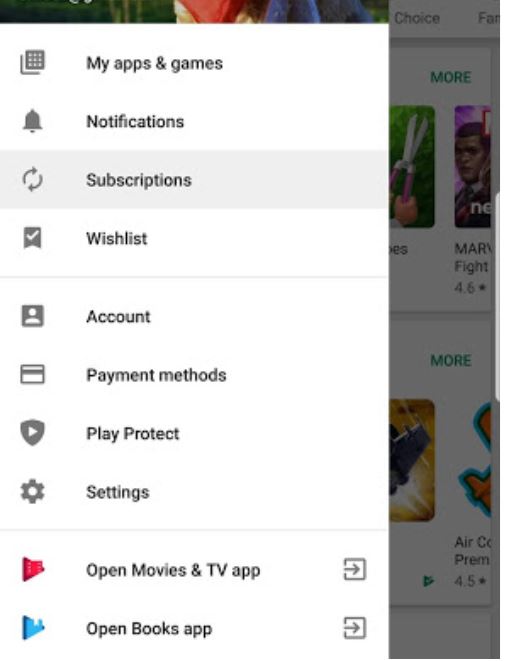The image features a tablet, likely an iPad or Galaxy Tab, displaying an app store interface. On the right edge of the screen, there's a faint gray line positioned near the middle. The background area shows the app store, showcasing various apps with images and partially visible titles. One of the displayed app ratings reads 4.6 with a star next to it.

On the left side of the screen, there's an overlay menu listing: "My Games and Apps," "Notifications" with a bell icon, "Subscriptions" with two circular arrows, "Wish Lists" with a banner and checkmark, "Account," "Payment Methods," "Play Protect," "Settings," "Open Movies and TV App," and "Open Books App". Each menu item has a corresponding icon, with the "Open" sections featuring colorful icons, and boxes with right-pointing arrows. This detailed interface highlights the tablet's organizational layout for managing apps and settings.